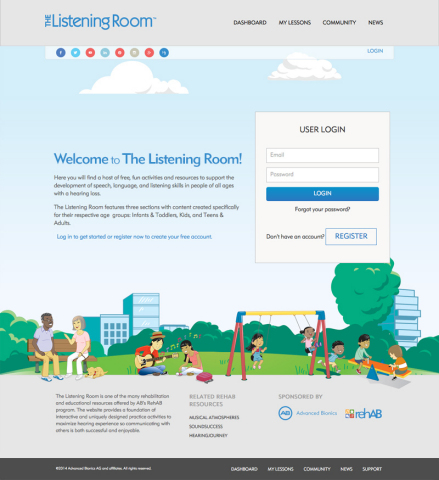The image features a webpage from a website called "The Listening Room." On the left side of the page, beside an owl illustration, the text "The Listening Room" is written sideways and is trademarked. To the right of the owl, in uppercase black letters, "DASHBOARD" is prominently displayed, followed by sections labeled "MY LESSONS" and "COMMUNITY NEWS."

Below these sections, there's a light blue clickable box, though its contents are not easily readable. Adjacent to this, a dark blue icon representing Facebook, along with other icons in light blue, red, and greenish-blue, follow in sequence. On the far right is a "LOGIN" option in blue.

The background of the webpage features a sky with white, puffy clouds designed in a clip-art style. Towards the bottom, there is an illustration of various people in a park setting. This includes a white woman sitting on a park bench with her dog, holding the leash, and a black man. Government buildings and trees fill the background. There's also a musician playing guitar for a girl, people on swings, and a child running near a seesaw.

Above this park scene is a user login box where users can enter their email and password, with a blue "LOGIN" button below it, along with a "Forgot Your Password?" link. For new users, there's a "Register" button that is transparent. The left side of the page contains a "Welcome to The Listening Room" message in blue text, followed by a description of the website. It also mentions that the site is sponsored by REHAB and Advanced Bionics.

At the webpage's bottom, similar navigation options are repeated: "DASHBOARD," "MY LESSONS," "COMMUNITY NEWS," and "SUPPORT." There's also the trademark information displayed at the bottom left.